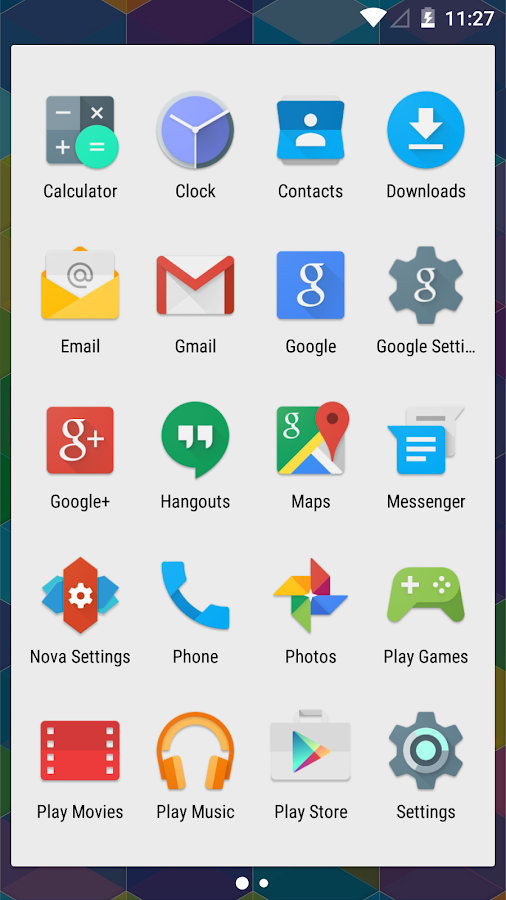A screenshot from a mobile device or tablet displaying the home screen. In the top-right corner, there is an indicator showing full Wi-Fi connectivity without any cellular service. The battery icon reveals a low charge, around 20%, and it is currently charging. The timestamp at the top indicates that the screenshot was taken at 11:27.

The home screen contains multiple app icons arranged in a 4x5 grid pattern. The first row consists of Calculator, Clock, Contacts, and Downloads apps. The second row includes Email, Gmail, Google, and Google Settings, denoted by a gear icon. The third row features Google+, Hangouts, Maps, and Messenger apps. The fourth row contains Nova Settings, Phone, Photos (represented by a colorful pinwheel), and Play Games apps. The fifth and final row includes Play Movies, Play Music, Play Store, and the general Settings app.

Given the substantial presence of Google applications like Gmail, Google+, Google Hangouts, Google Maps, and Google Photos, it is likely that this is a Google device. Other notable apps include the Messenger app and the Play Store, further indicating the device's integration into the Google ecosystem.